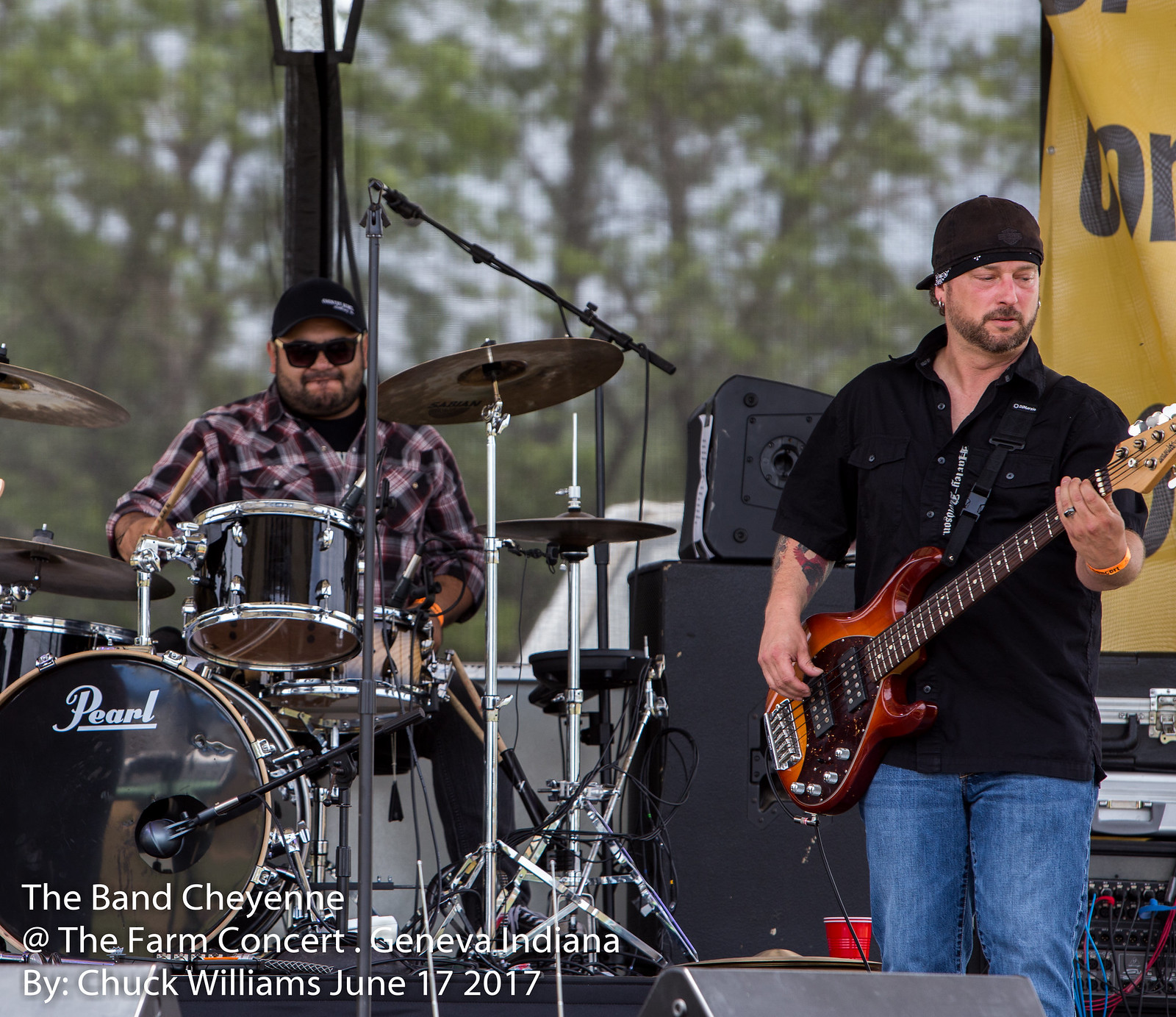This photograph captures a close-up view of two musicians performing on an outdoor stage at the Farm Concert in Geneva, Indiana, featuring the band Cheyenne. The image, taken by Chuck Williams on June 17, 2017, prominently displays the band's name in the lower left-hand corner. On the left, a drummer is seated behind a large drum set labeled "Pearl," dressed in a purple checkered flannel shirt, gray sunglasses, a black baseball cap, and sporting a beard and mustache. On the right, a guitarist stands wearing a black button-up shirt, black cap worn backwards, and blue jeans. The guitarist's left hand sports a ring on the ring finger, possibly a wedding ring, and he holds a brown and black five-string guitar. In the background, a partially visible yellow banner with black lettering hangs, though its text is obscured. The setting is an open-air stage surrounded by tall, green trees, adding a natural backdrop to the performance. Dominant colors in the image include black, white, brown, orange, and blue, with details such as monitor speakers and a red plastic cup adding to the scene's immersive atmosphere.